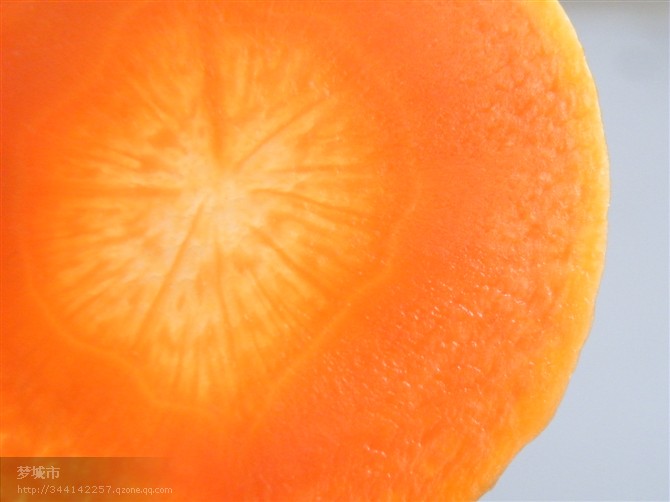The image appears to be a close-up photograph of a peach-colored fruit, likely an orange. The fruit's surface, which almost entirely fills the image, is characterized by a gradient of color that transitions from dark orange at the periphery to a lighter, almost translucent orange at the center. This central area, resembling a core, radiates straight lines outward like sun rays towards the edges. Although predominantly orange, the upper right portion of the image features a light gray segment expanding downward and widening at the bottom right. At the bottom left corner, faint white writing, possibly Asian characters followed by numbers, is visible. The fruit's texture appears fuzzy, adding to its detailed and vivid representation.